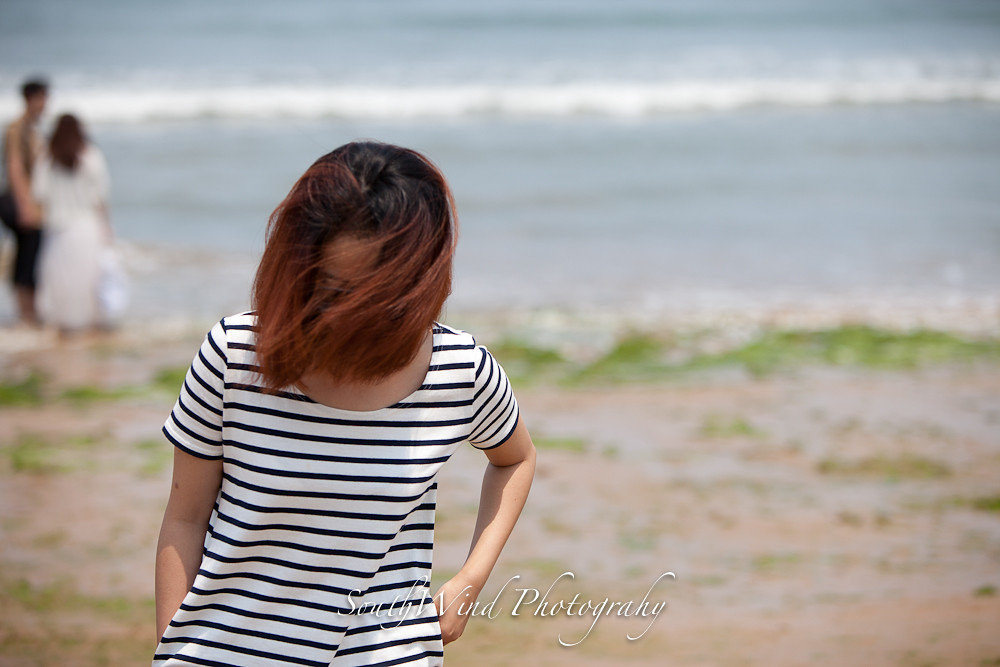A photograph captures a serene beach scene featuring a woman standing prominently in the foreground. The background is softly blurred, accentuating the calm, low waves of the ocean and patches of greenery on the sandy shore. The woman, wearing a black and white striped short-sleeved t-shirt, has her right arm in her pocket and her left arm partially raised, seemingly toward her pocket. Her hair, a striking blend of black roots transitioning to burgundy ends, is being blown across her face by the wind, obscuring her facial features. She wears glasses, adding an intriguing detail to her appearance. In the blurred background, a couple can be seen standing near the waterline. The man, in jeans and a white shirt, is visible in profile, holding hands with a woman in a white dress. Centered at the bottom of the photograph is the text "South Wind Photography," elegantly scripted in white cursive.